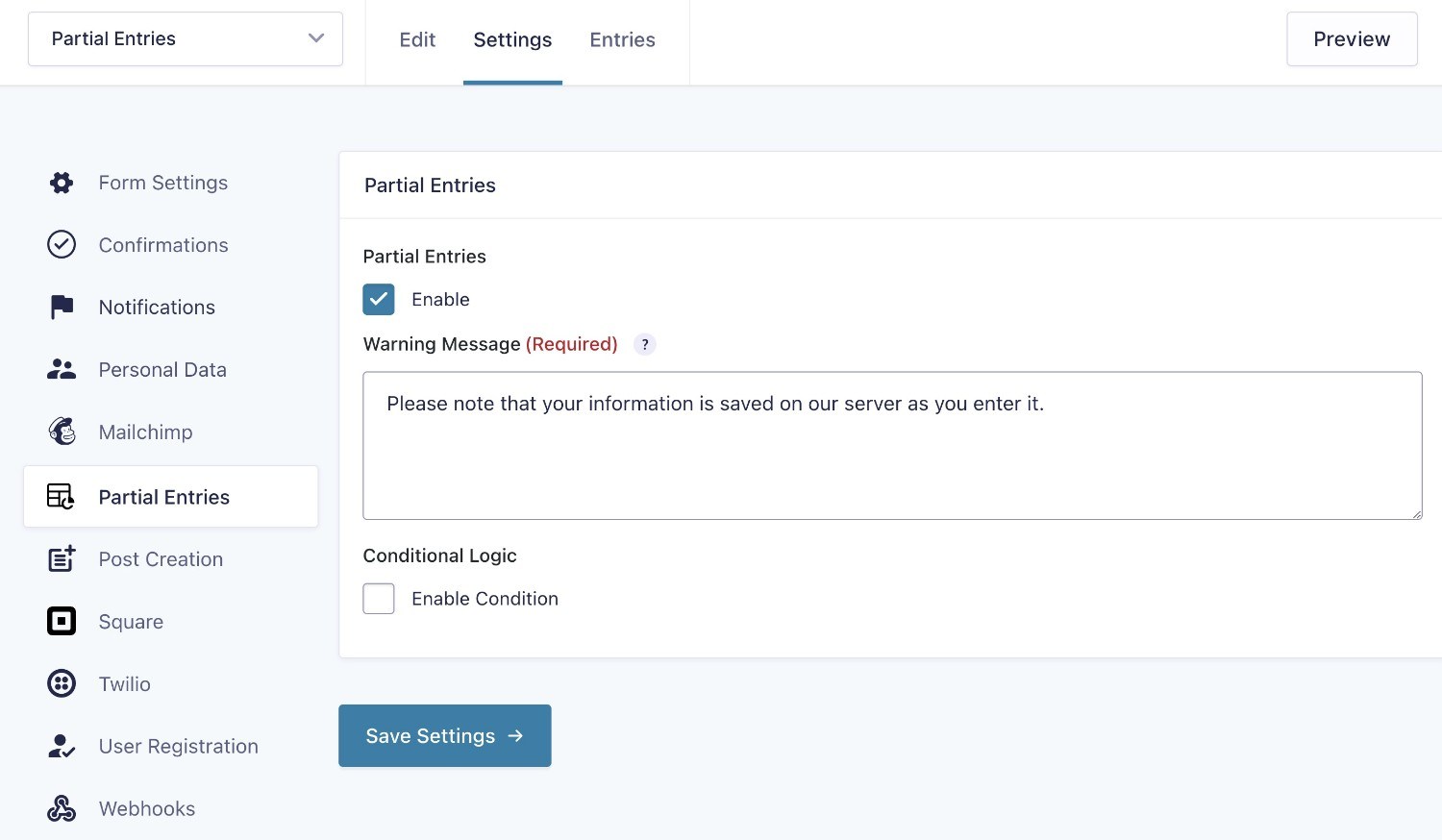Screenshot of a Website Editing Program Interface:

This image is a screenshot of a web editing program interface, likely used for managing forms and entries. The top left corner of the interface features a label "Partial Entries" with an adjacent drop-down menu for additional options. Situated to the right are three tabs: "Edit," "Settings" (which is currently selected), and "Entries." On the far right, there is a prominent "Preview" button.

The left sidebar hosts a vertical menu with various configuration options, listed from top to bottom as follows: "Form Settings,” “Confirmations,” “Notifications,” “Personal Data,” “MailChimp,” “Partial Entries” (highlighted in white to indicate it's the active selection), “Post Creation,” “Square,” “Twilight,” “Twilio,” “User Registration,” and “Webhooks.”

The main content area under the active "Partial Entries" tab displays a configuration section with "Partial Entries" prominently at the top. This feature appears to be enabled, as indicated by a checked checkbox. Below this, there is a warning message in red text, reading "Required" within parentheses. The entered warning message states: "Please note that your information is saved on our server as you enter it." Further down, there is an option for "Conditional Logic" with the ability to enable conditions, though this option is currently unchecked.